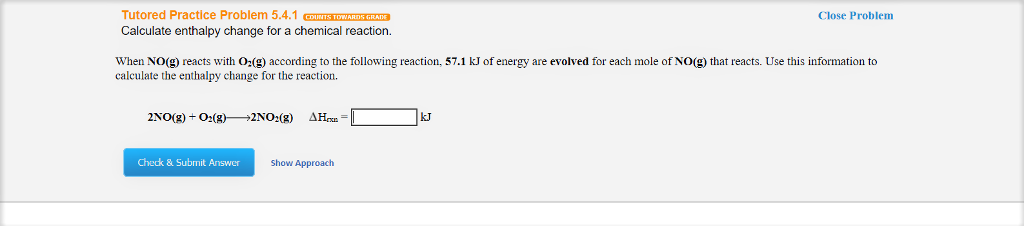This is a detailed and descriptive caption for the given image:

The partial screenshot depicts an educational interface with a gray and light gray background and a rectangle with a darker gray outline. At the top of the rectangle, in prominent orange text, it reads "Tutored Practice Problem 5.4.1." Adjacent to this, a small orange banner with white text states "Counts toward grade." On the upper right-hand corner of the rectangle, there is blue text that says "Close Problem."

Below the heading, black text instructs users: "Calculate the enthalpy change for the chemical reaction. When NO(g) reacts with O2(g) according to the following reaction, 57.1 kJ of energy are evolved for each mole of NO(g) that reacts. Use this information to calculate the enthalpy change for the reaction."

The instruction is followed by a space for input: a chemical formula, an equal sign, and a blank box designated for the user’s answer. Directly beneath this input area, a blue button with white text encourages action with the prompt "Check and Submit Answer." Next to this button, blue text provides an optional hint with the words "Show Approach."